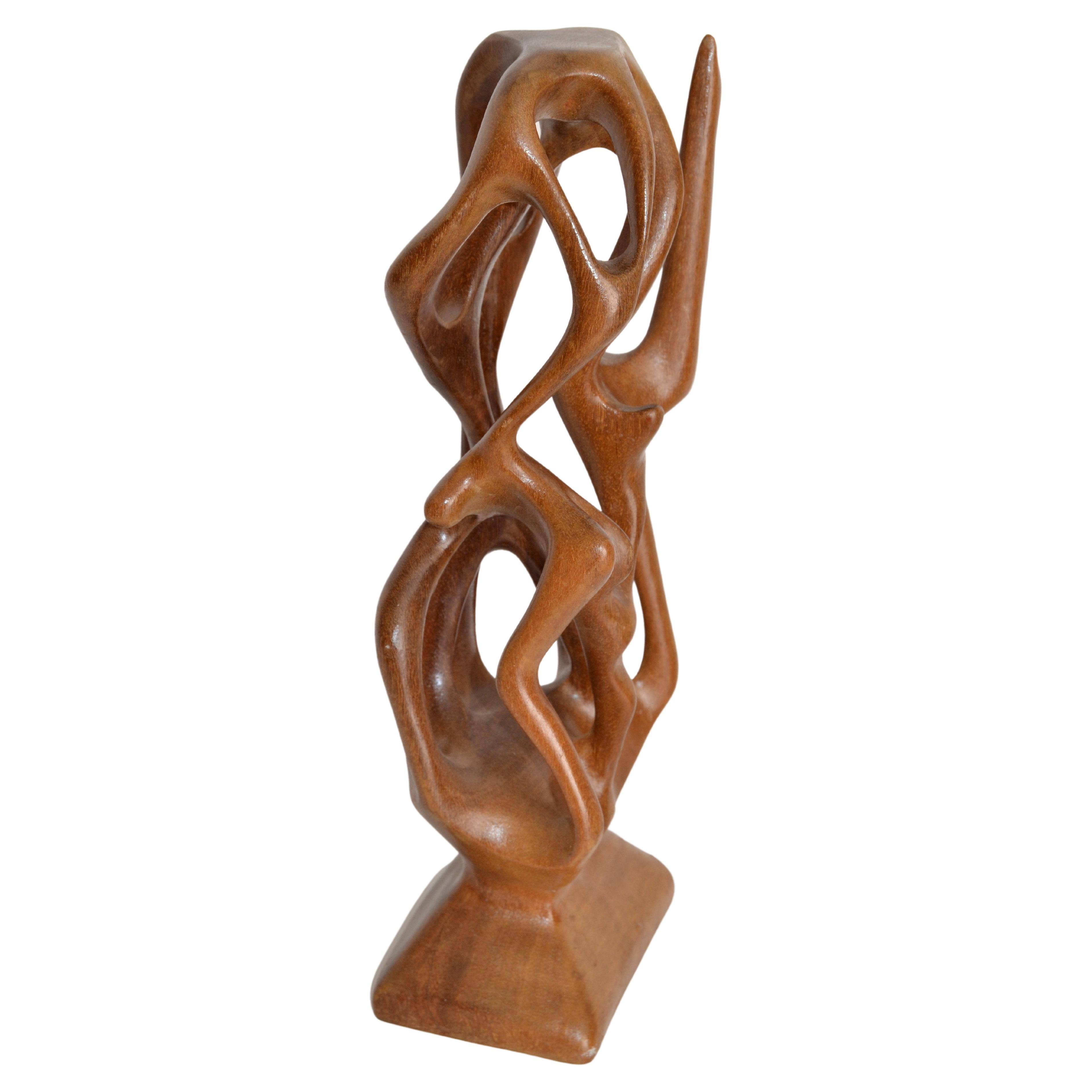The image showcases a tall, intricately carved wooden statue, approximately 8 to 10 inches high, rendered in rich brown wood that might be oak or chestnut. This abstract piece features an array of sensuous curves and hollow loops, creating a wiry, almost ornamental design that evokes the elegant contours of a svelte figure. The statue's texture boasts a caramel-like sheen, enhancing its aesthetic appeal. Notably, the top of the statue is adorned with a stick-like, pointy object projecting upwards, while its upper left side maintains a flat surface. The lower part of the statue gradually tapers from a square base to a more pyramid-like shape, from which the intricate carvings and patterns emanate, including thin sections and holes that contribute to its airy, light-filled structure.